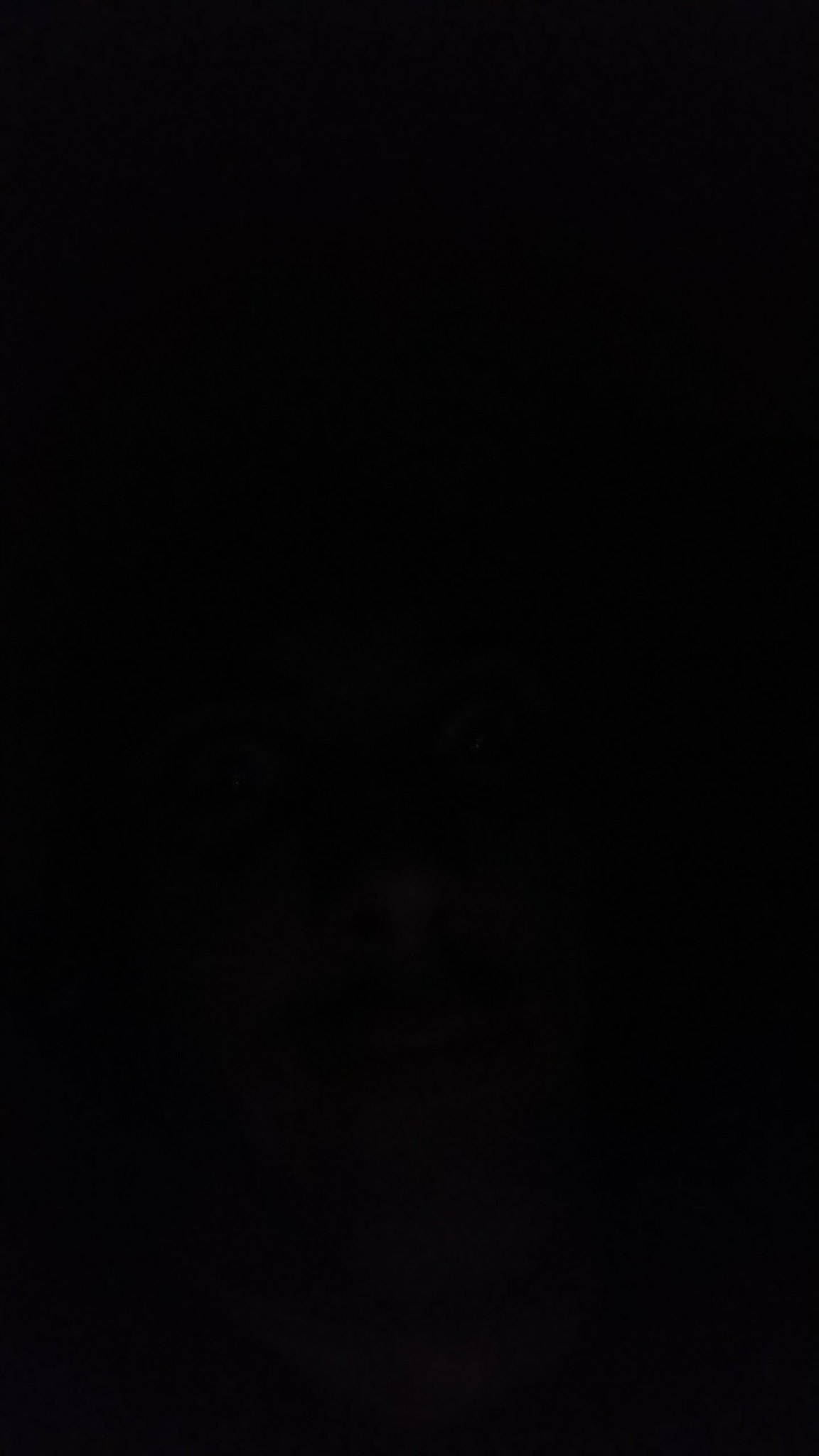The photograph is a vertically aligned, rectangular selfie taken in an extremely dark environment, predominantly black with barely visible details. The image, nearly pitch black, features a man's face faintly visible in the middle and lower portion. Despite the darkness, you can discern his wide-open eyes, a very thin mustache without a beard, and slightly open mouth revealing a hint of his teeth. The sides of his face are shrouded in darkness, and only a subtle outline of his neck and shirt collar can be made out against the inky black background.